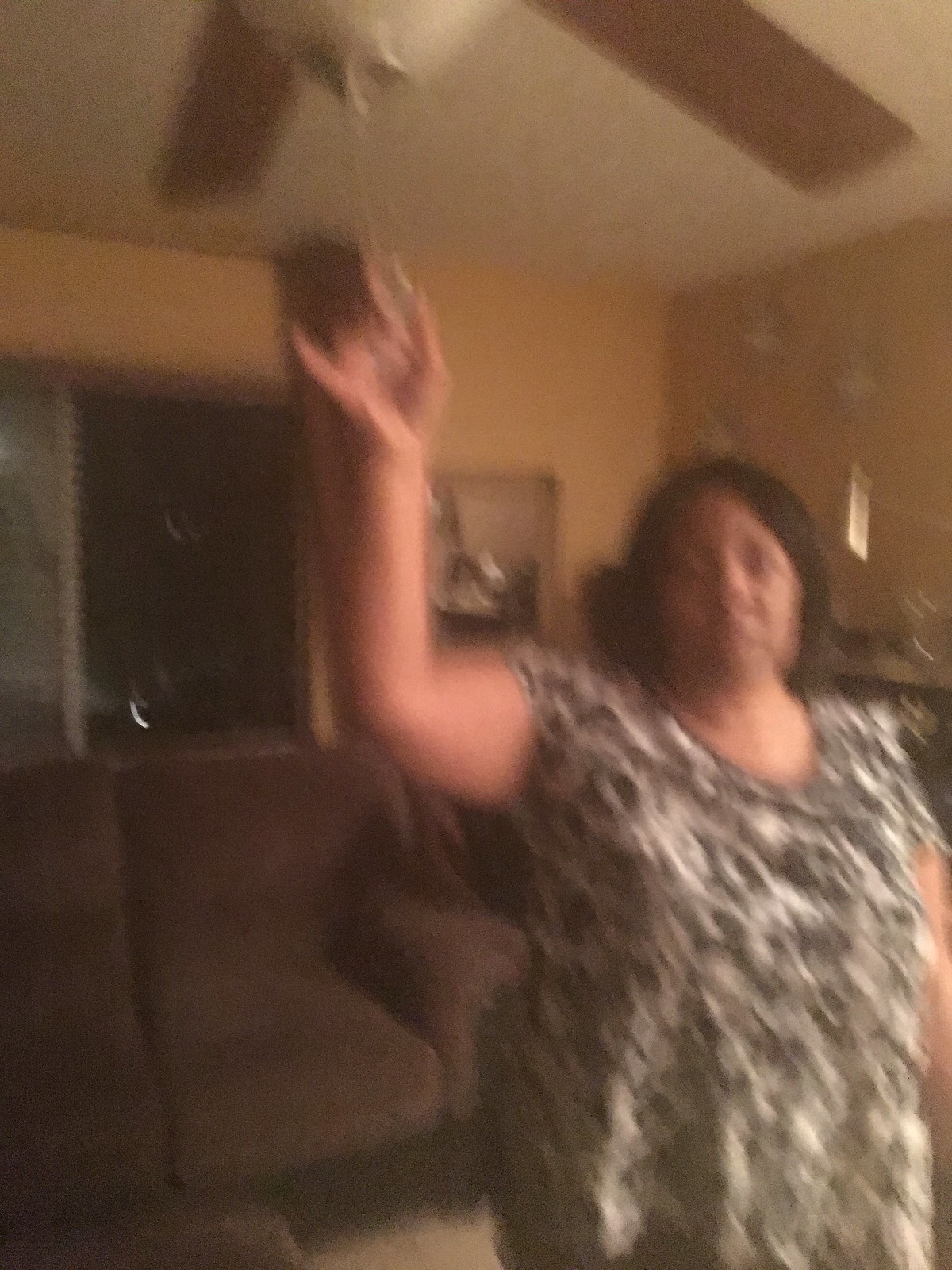In this very blurry, low-resolution image, we see an African-American woman standing in a living room. She is slightly overweight and wearing a short-sleeved, black-and-white muumuu-style dress. The woman is facing the camera, positioned in the lower right corner of the photo, with her right arm raised, possibly waving or reaching for the chain switch of the ceiling fan above her. The fan has brown blades and a white globe light fixture, set against a white ceiling.

The living room features a dark brown two-piece sofa in the background, and the walls are painted a yellowish-tan color, adorned with some indiscernible decor and an art piece that is situated in a nook. There is also an open patio door or window, revealing the blackness of night outside, adding to the indoor ambiance. The image's blurriness makes it difficult to ascertain her exact mood or precise gestures.